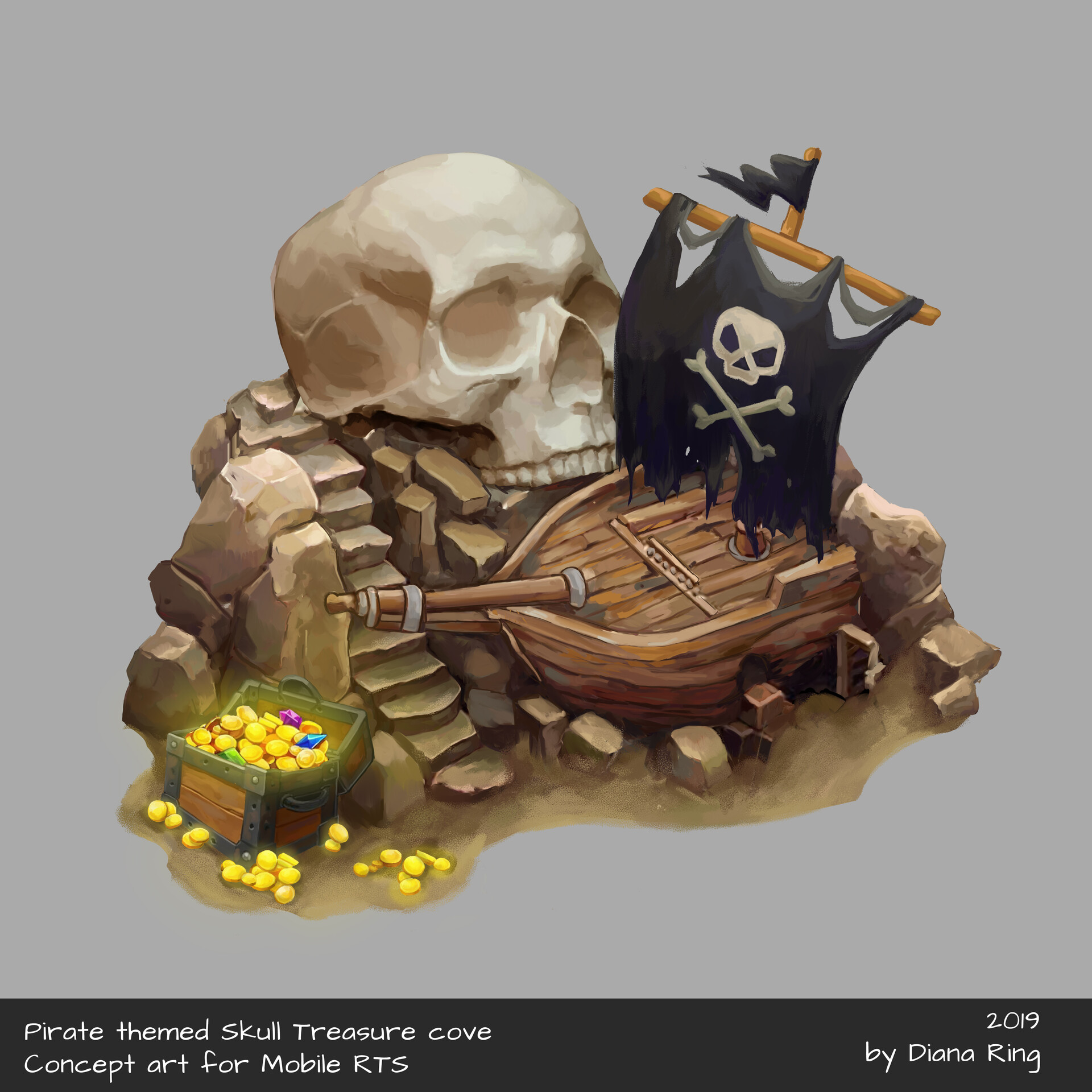This detailed digital artwork, titled "Pirate Themed Skull Treasure Cove Concept Art for Mobile RTS," is by Diana Ring, created in 2019. In the center of the light gray background, the scene depicts the front half of a wooden pirate ship, which has sunk and crashed into an imposing temple adorned with a large stone skull. The pirate ship prominently features a black flag with a white skull and crossbones. A staircase ascends from the wreckage to the eerie skull temple. At the base of the stairs, there is a treasure chest spilling over with gold coins and vibrant jewels in green, magenta, and blue. This concept art is framed by a thin black band at the bottom, containing white text that provides the title and the artist's information, making up approximately one-tenth of the image's height. The overall composition powerfully evokes a sense of mystery and adventure, encapsulating the pirate theme perfectly.